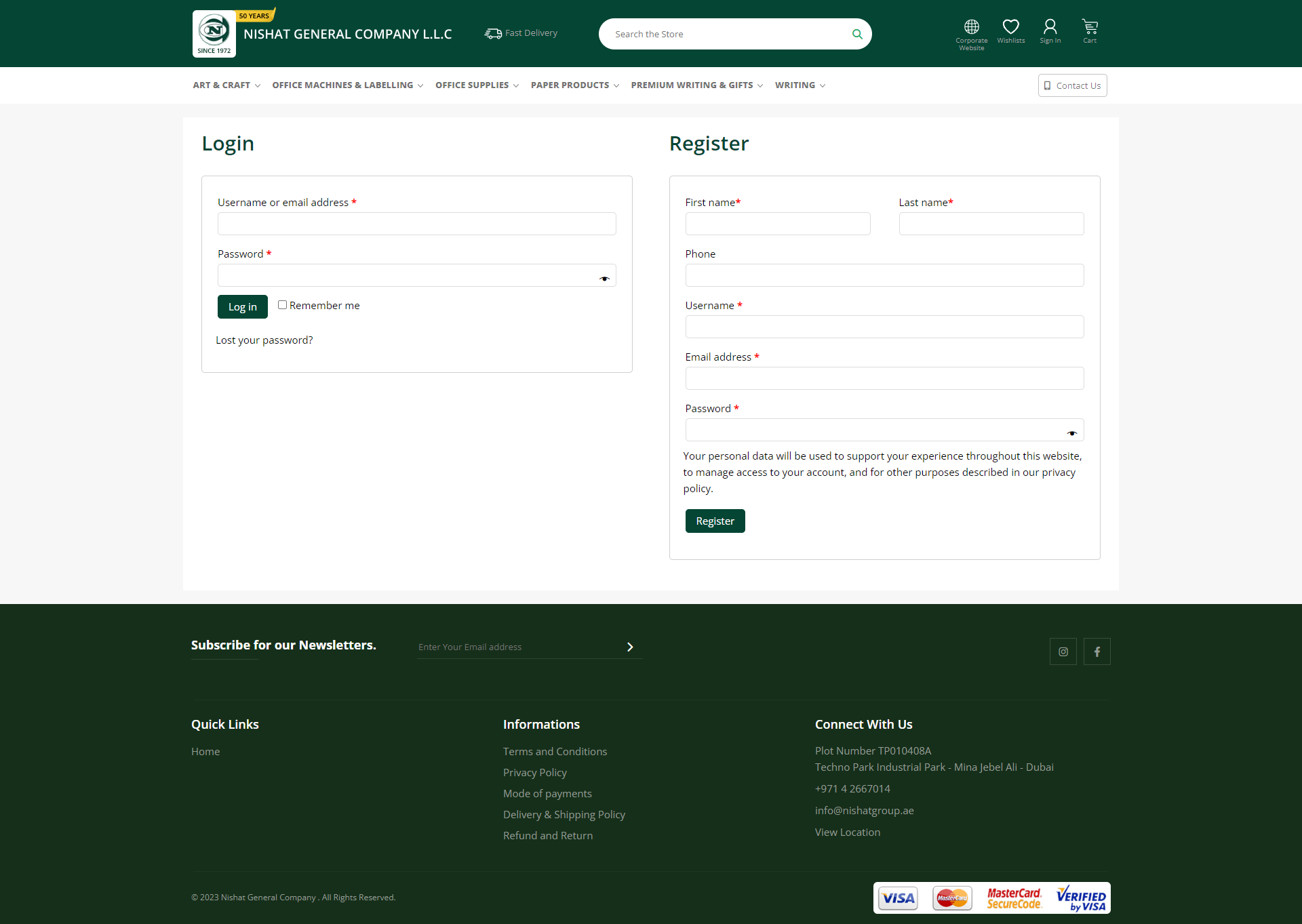The image features the homepage of Nishat Central or General Company, LLC, presented with a clean, white background. At the top, there is a prominently displayed search bar accompanied by a magnifying glass icon on the right. Adjacent to the search bar are a series of icons: a globe, a heart, a user profile, and a shopping cart.

Below, a navigation menu lists several categories: "Art and Craft," "Office Machines and Labeling," "Office Supplies," "Paper Products," "Premium Writing," and "Gifts and Writing."

The page also includes a login area with fields labeled "Username or Email Address" and "Password," both featuring red asterisks indicating required information. The login button is styled as a green rectangle with white text.

Additional options under the login include a checkbox for "Remember Me" and links for "Lost your password?" and "Register."

The registration section includes fields for "First Name," "Last Name," "Username," "Email Address," and "Password," all marked with red asterisks. The register button is also a green rectangle with white text.

At the bottom of the page, a green subscription bar invites users to "Subscribe for our newsletters." Quick links are provided for easy navigation, including "Home," "Information," "Terms and Conditions," and "Privacy Policy."